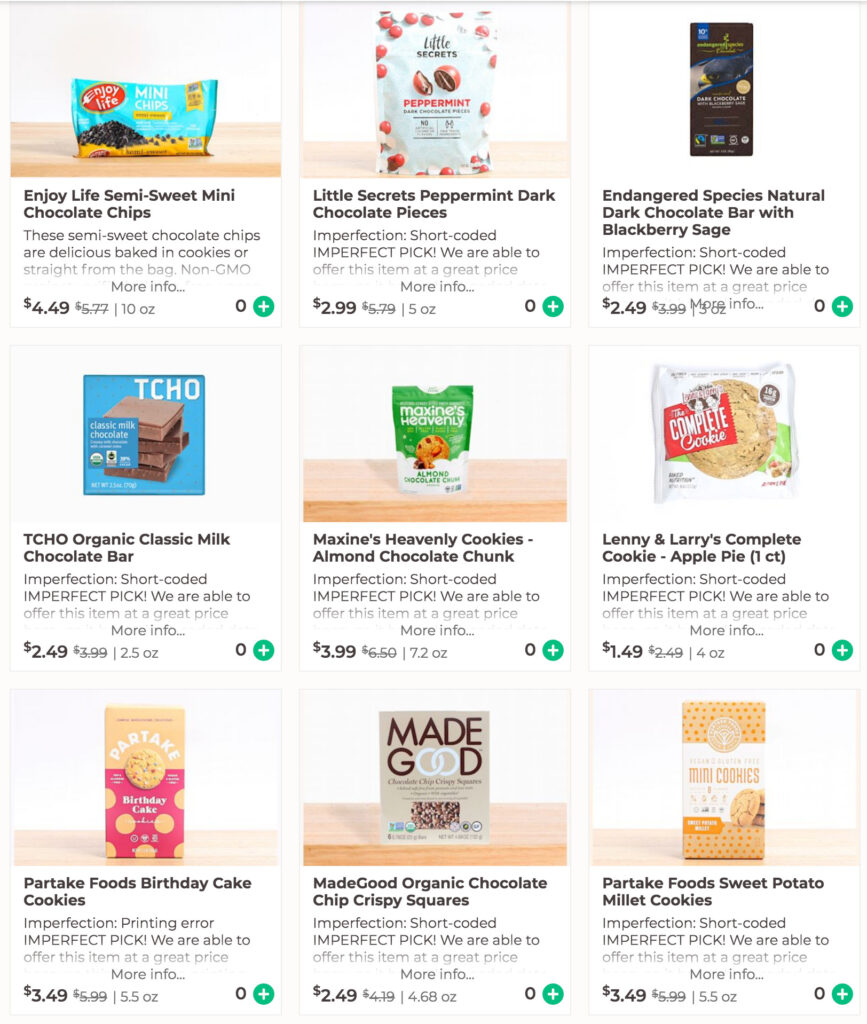The web page features a variety of items, predominantly different types of chocolate and cookies, each displayed with detailed descriptions, prices, and specials:

1. **Enjoy Life Semi-Sweet Mini Chocolate Chips**  
   - **Image Description**: A bag of chocolate chips with a cyan blue background. The packaging features a red circle with a fork icon and the words "Enjoy Life" and "Mini Chips" in black text.
   - **Text Details**:  
     - Bold black text: "Enjoy Life Semi-Sweet Mini Chocolate Chips." 
     - Regular black text: "These semi-sweet chocolate chips are delicious baked in cookies or straight from the bag. Non-GMO."
     - Price: $4.49 (previously $5.77)
     - Quantity: 10 ounces
     - Green circle with white plus sign indicating zero quantity. 

2. **Little Secrets Peppermint Dark Chocolate Pieces**  
   - **Image Description**: Peppermint dark chocolate pieces. The packaging emphasizes "Little Secrets."
   - **Text Details**:  
     - Bold black text: "Little Secrets Peppermint Dark Chocolate Pieces." 
     - Gray text: "Imperfection, short coded imperfect pick. We are able to offer this item at a great price."
     - Price: $2.99
     - Quantity: 5 ounces
     - Green circle with white plus sign indicating zero quantity. 

3. **Endangered Species National Dark Chocolate Bar with Blueberry Sage**  
   - **Image Description**: A close-up image of a special dark chocolate bar by Endangered Species, indicating a cause for raising money for endangered species.
   - **Text Details**:  
     - Bold black text: "Endangered Species National Dark Chocolate Bar with Blueberry Sage." 
     - Gray text: "Imperfection, short coded imperfect pick. We are able to offer this item at a great price."
     - Price: $2.49 (previously $3.99)

4. **TCHO Organic Classic Milk Chocolate Bar**  
   - **Image Description**: Light and dark brown chocolate bars with the brand name "TCHO" in white text and "Classic Milk Chocolate" in dark blue.
   - **Text Details**:  
     - Bold black text: "TCHO Organic Classic Milk Chocolate Bar."
     - Gray text: "Imperfection, short coded imperfect pick. We are able to offer this item at a great price."
     - Price: $2.49 (previously $3.99)
     - Quantity: 2.5 ounces

5. **Maxine's Heavenly Almond Chocolate Chunk Cookies**  
   - **Image Description**: A dark green bag containing brown cookies with almonds.
   - **Text Details**:  
     - Bold black text: "Maxine's Heavenly Almond Chocolate Chunk Cookies."
     - Price: $3.99 (previously $6.50)
     - Quantity: 7.5 ounces

6. **Lenny & Larry's Complete Cookie Apple Pie**  
   - **Image Description**: A giant brown cookie inside a white bag.
   - **Text Details**:  
     - Bold black text: "Lenny & Larry's Complete Cookie Apple Pie."
     - Price: $1.49 (previously $2.49)
     - Quantity: 4 ounces

7. **Partake Foods Birthday Cake Cookies**  
   - **Image Description**: A peach bag with red accents featuring images of cookies. The top text reads "Party Take" in bold white.
   - **Text Details**:  
     - Bold black text: "Partake Foods Birthday Cake Cookies."
     - Price: $3.49 (previously $5.99)
     - Quantity: 5.5 ounces

8. **Made Good Organic Chocolate Chip Squares**  
   - **Image Description**: Dark brown chocolate chip cookies.
   - **Text Details**:  
     - Bold black text: "Made Good Organic Chocolate Chip Squares."
     - Price: $2.49 (previously $4.19)
     - Quantity: 4.68 ounces

9. **Partake Foods Sweet Potato Millet Cookies**  
   - **Image Description**: Light brown and tan mini cookies in a bag with white and orange text, orange dots on a red background.
   - **Text Details**:  
     - Bold black text: "Partake Foods Sweet Potato Millet Cookies."
     - Price: $3.49 (previously $5.99)
     - Quantity: 5.5 ounces